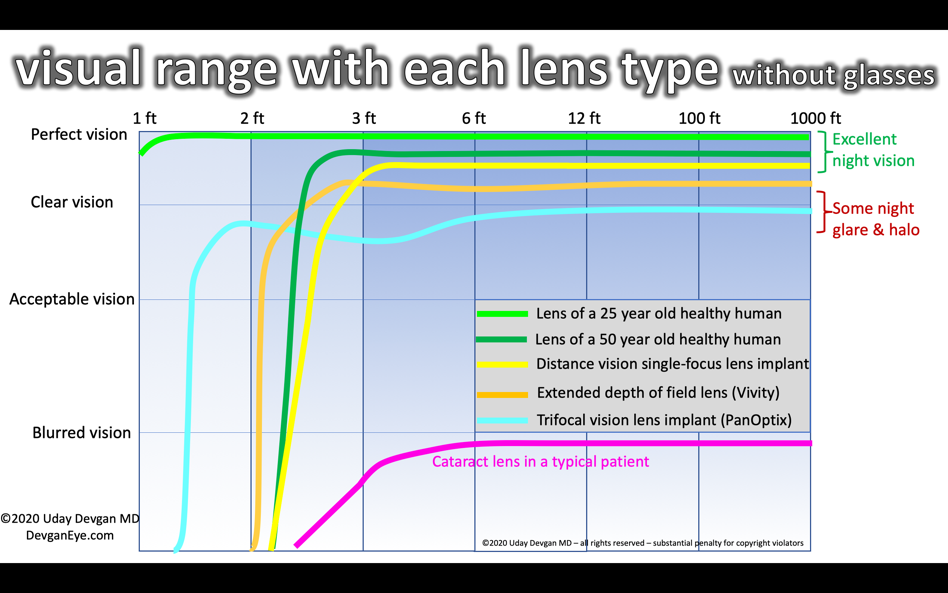The image is a detailed graph showcasing the visual ranges for different lens types compared to vision without glasses. Starting from the top, the graph classifies vision into four categories: perfect vision, clear vision, acceptable vision, and blurred vision. These categories are indicated by horizontal lines. The horizontal axis extends from 1 foot to 1,000 feet, while the vertical axis includes a footer noting, "Copyright 2020 Uday Devgan MD, devgan.com."

The perfect and clear vision tiers, marked in green, are labeled as "excellent night vision." This is contrasted with the light blue line representing trifocal vision, which notes "some night glare and halo." Different lens types are represented through various colored lines that curve and extend across the graph: 

- Light green indicates the visual range of a healthy 25-year-old human's lens.
- Dark green represents the lens of a healthy 50-year-old human.
- Yellow corresponds to a single-focus lens implant for distance vision.
- Orange depicts the extended depth of field lens.

Thin black stripes border the top and bottom of the graph, which has a white background and shades of blue within the chart itself. The key on the right-hand side decodes the color lines and their corresponding lens types, providing a clear visual comparison of the efficacy of each lens type across various distances.

Overall, this graph comprehensively shows how different lenses affect visual ranges, emphasizing how healthy human lenses at ages 25 and 50 outperform synthetic lenses in night vision and overall clarity.